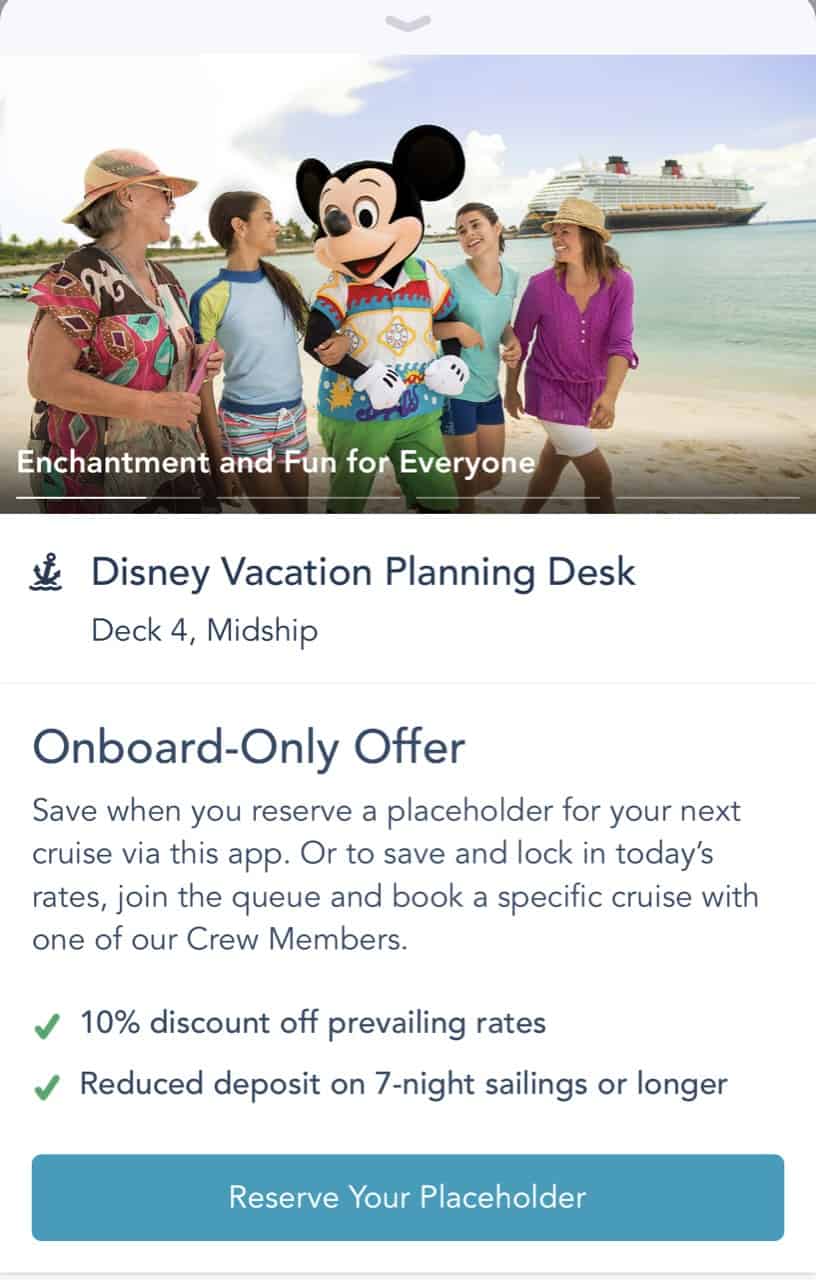**Descriptive Caption:**

The image depicts a vibrant and cheerful Disney vacation planning desk advertisement. In the background, a picturesque scene of a family on a beach is shown. Two women and two young girls, all dressed in colorful outfits, walk arm in arm with Mickey Mouse, who is wearing a multicolored shirt. Behind them, a majestic cruise ship can be seen against a beautiful beach backdrop, creating a sense of magical adventure.

The overlay text on the image reads "Enchantment and Fun for Everybody," emphasizing the inclusive and joyous nature of Disney vacations. Below this, there is additional informational text that states "Disney Vacation Planning Desk, Deck 4 Midship." The ad highlights the exclusive onboard-only offer, communicating, "Save when you reserve a placeholder for your next cruise via this app or to save and lock in today's rates, join the queue and book a specific cruise with one of our crew members."

Further down, the ad lists enticing benefits with green check marks for easy identification, including "10% discount off prevailing rates" and a "Reduced deposit on seven-night sailings." At the bottom, a call-to-action in an appealing teal blue color encourages viewers to "Reserve Your Placeholder," inviting them to plan and secure their next Disney cruise experience.